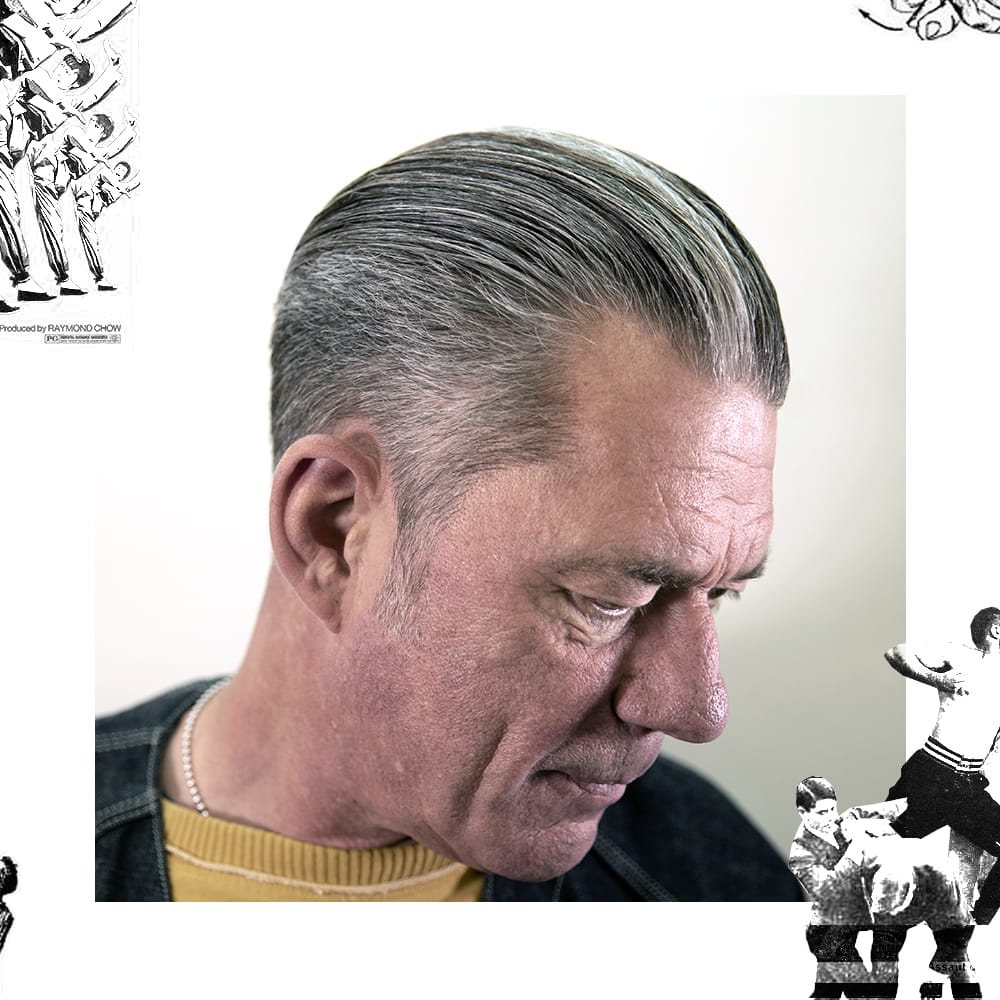The photograph captures a close-up of a serious, solemn-looking Caucasian man in his 50s or 60s with dark hair generously streaked with silver and white, combed or slicked back. He gazes downward toward the bottom right corner of the image. He is wearing a mustard yellow crewneck sweater or shirt, partially concealed by a dark-colored jacket. A metal ball chain necklace is visible around his neck. The photo is bordered with what appears to be black and white images and illustrations from a bygone era, including historic or sport-themed photos, possibly of boxing or baseball, and one showing figures engaged in martial arts. These smaller images frame the main picture decoratively, adding a nostalgic and historical layer to the composition.